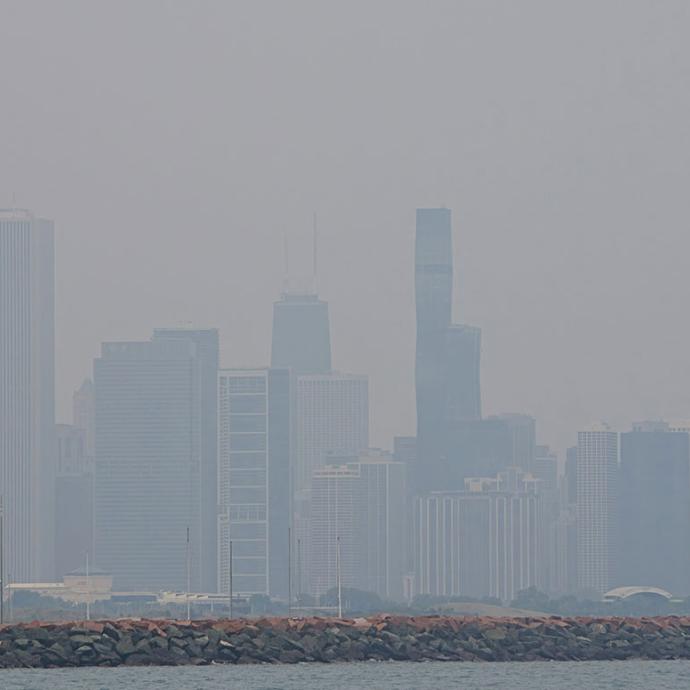This full-color photograph, taken outdoors during the day in natural light, captures a panoramic view of a city skyline veiled in thick smog or mist, rendering the sky and buildings a pervasive gray color. The image, which is vertically rectangular, showcases an expanse of water in the lower part, appearing grayish likely due to the overcast atmosphere. Bordering this water body is a rocky shoreline composed of dark grey and brown stones and black boulders stacked on top of each other. Beyond the shore, numerous skyscrapers of varying heights loom in the background, their cuboidal forms barely discernible through the heavy haze. The overall effect suggests either dense fog or severe pollution, obscuring much of the architectural detail.